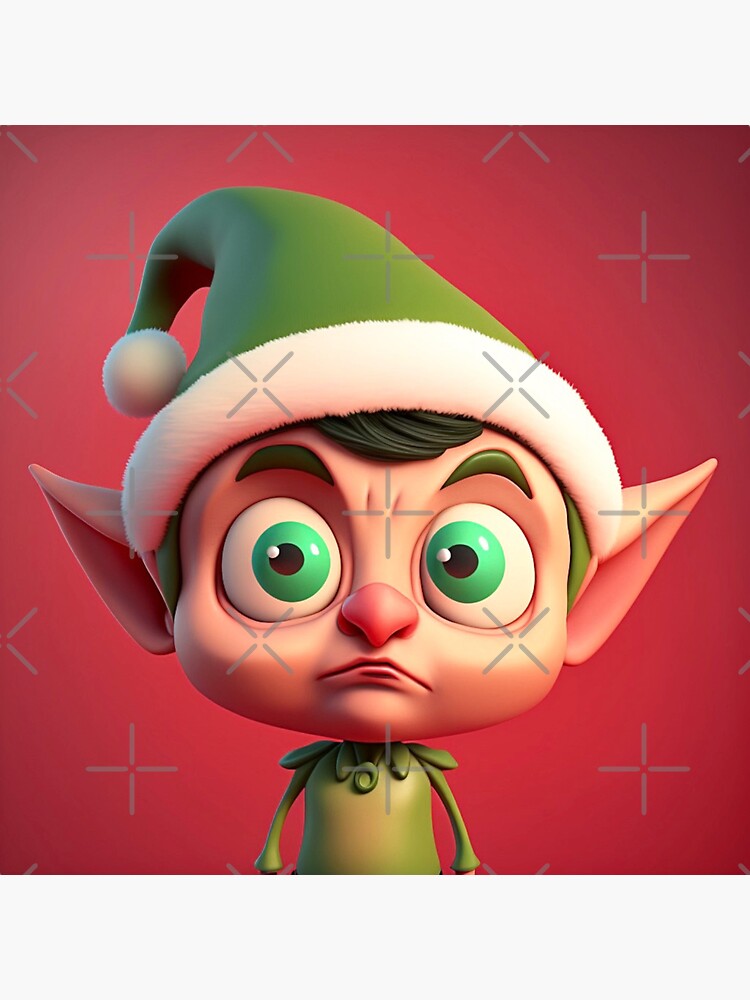This is a computer-animated image of what appears to be an angry elf set against a red background that fades from darker on the edges to lighter in the center. The background features a pattern of light gray plus signs and X's, possibly as watermarks, arranged in rows across the image. The elf has exaggerated wide, almost egg-like eyes with bright green irises, dark green pupils, and tiny white highlights. His facial features include a prominent red nose and downturned mouth, giving him an angry expression. The elf's hair and eyebrows are dark green. He's wearing a green suit and a green Santa hat with a white furry brim and a white puffball at the tip, which slightly transitions to blue in a gradient. His ears are pointy, completing the characteristic elf look.